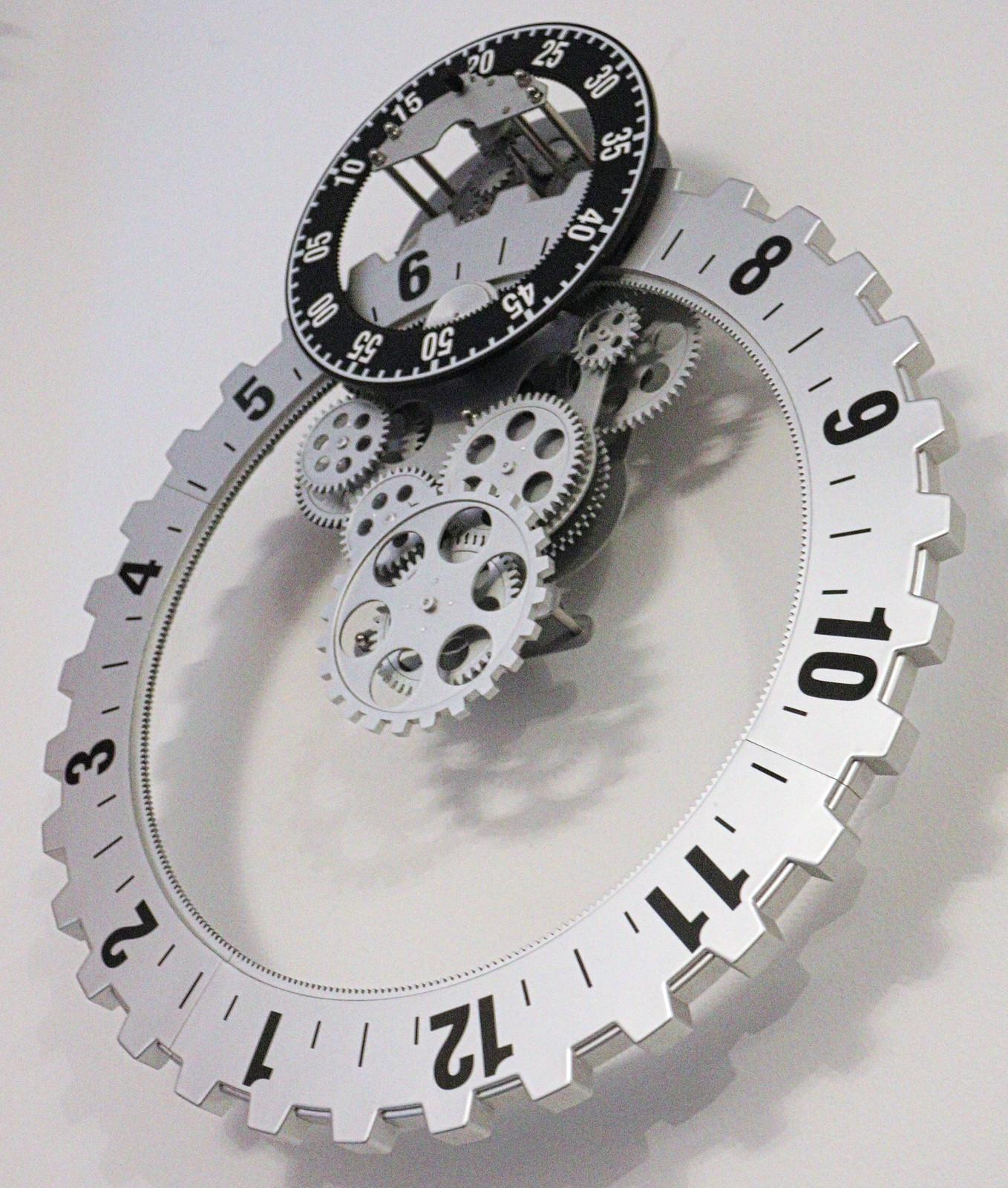The image showcases a detailed close-up of a complex mechanical device, resembling the intricate inner workings of a timepiece or precision instrument. Dominating the composition is a large silver component engraved with black numerical markings ranging from 1 to 12. Surrounding this principal piece are several notches that contribute to its elaborate design. Centrally located is a sophisticated mechanism composed of intermeshing gears and other metallic elements, exuding a sense of meticulous engineering. Above this mechanism is a black circular element, featuring white numerical indicators and tiny notches. The numbers on this circle start at '00' and incrementally increase up to '55', suggesting a measure of time or degree. The combination of black and silver hues with precise detailing underscores the technical and functional nature of the device.